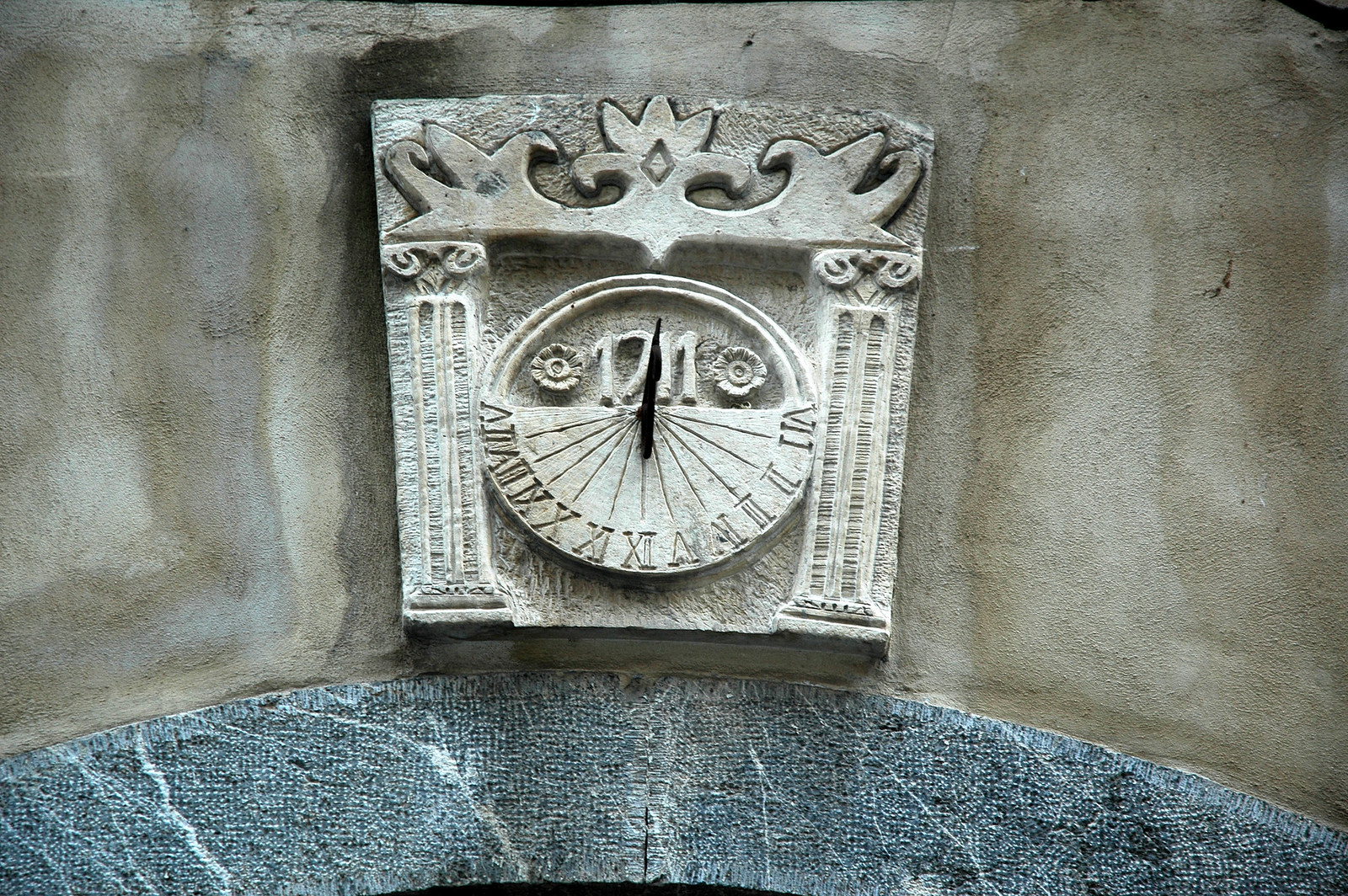A vibrant color photograph captures an intricately carved architectural detail on an aged stone building. The central feature, roughly square with an elegant curve at the top, showcases exquisite scrollwork carved into the stone. Flanking this section are two slender pillars, one on the left and one on the right, adding to the grandeur. Dominating the center is a striking clock adorned with Roman numerals, a timeless focal point. The backdrop consists of weather-beaten stone walls in a palette of grays and browns, marked by the passage of time. Beneath this ornate area, an arch frames what appears to be a window or doorway, distinguished by its bluish-gray marble-like surface, further enhancing the architectural splendor.